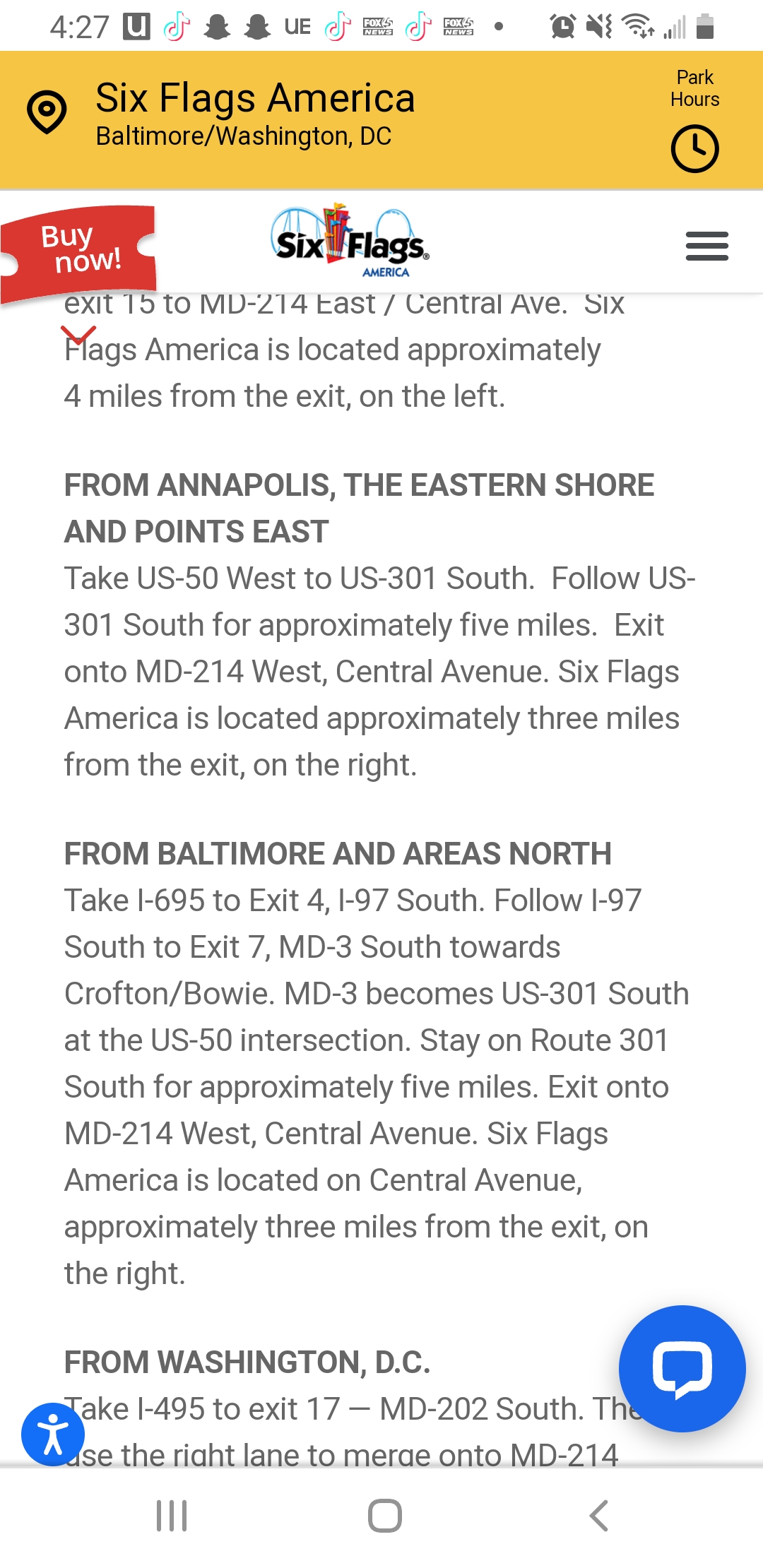The image is a screenshot taken on a smartphone, showcasing a variety of elements on the screen. At the very top, there is a white notification bar filled with several icons and details. From left to right, it displays the time "4:20", followed by a darker square containing a white "U". Next to it is the white TikTok logo, then two icons resembling Snapchat's bell symbol, and the letters "EU". Further along, there is another TikTok logo, a series of two grey rectangles, another TikTok logo, the rectangles again, a small dot, a darkly colored alarm clock icon with white hands, a volume icon with a speaker pointed to the right and a line through it indicating vibrate mode, a full WiFi symbol, a phone signal indicator showing two bars, and finally, a half-full battery icon.

Below this notification bar is a yellowish banner with black text that reads "Six Flags America, Baltimore/Washington D.C." To the right of this text, it says "Park Hours" accompanied by a black clock icon. The rest of the page is white with various details. In the upper left corner, there is a white ticket-shaped icon with the text "Buy Now". Below this icon, the Six Flags logo is displayed in black, with "America" written underneath. The main section of the screenshot contains a large block of text providing directions to the park, depending on the traveler's starting location.